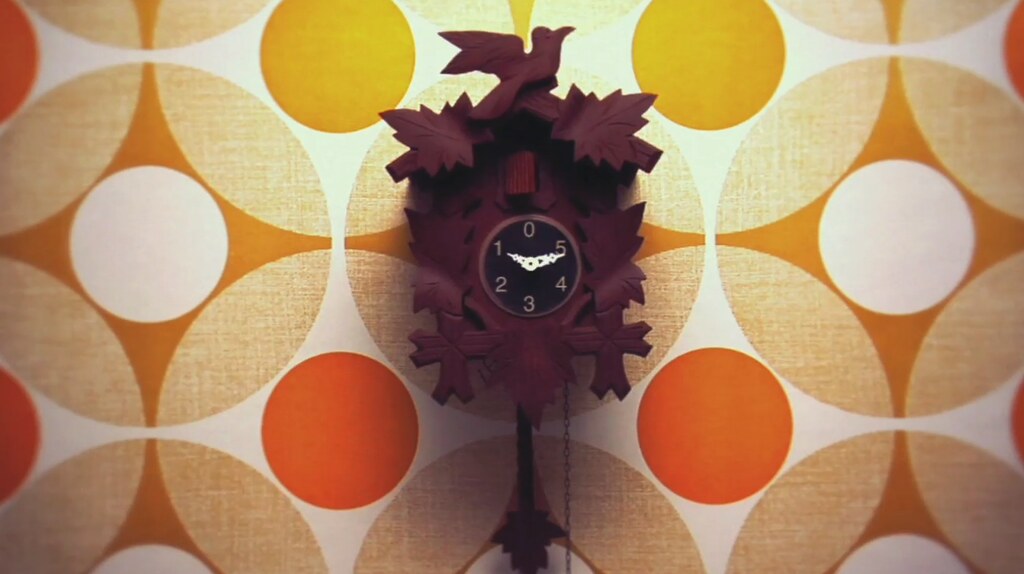This image features a stylized and ornate cuckoo clock centrally mounted on a wallpapered wall. The cuckoo clock, possibly a computer graphic, has a detailed design reminiscent of a birdhouse, with a burgundy, solid wood-like appearance. The clock has a triangular roof and a rectangular body adorned with intricately carved leaves and a small bird perched at the peak looking upwards. The face of the clock is a black circle with stylized white hands and numbers arranged in an unconventional pattern reading 0, 5, 4, 3, 2, 1 clockwise. A small, partially open door is located above the clock face, where the cuckoo bird would emerge. Below the clock face, a pendulum hangs down, adding to its classic charm. 

The background wallpaper features a distinct 70s-style pattern of overlapping circles in shades of orange, yellow, tan, and white. The circles are large with white centers and are bordered by a radial design of four semicircles positioned at each corner, creating a dynamic, retro aesthetic. This setting provides a vibrant and nostalgic backdrop to the cuckoo clock's refined detail.